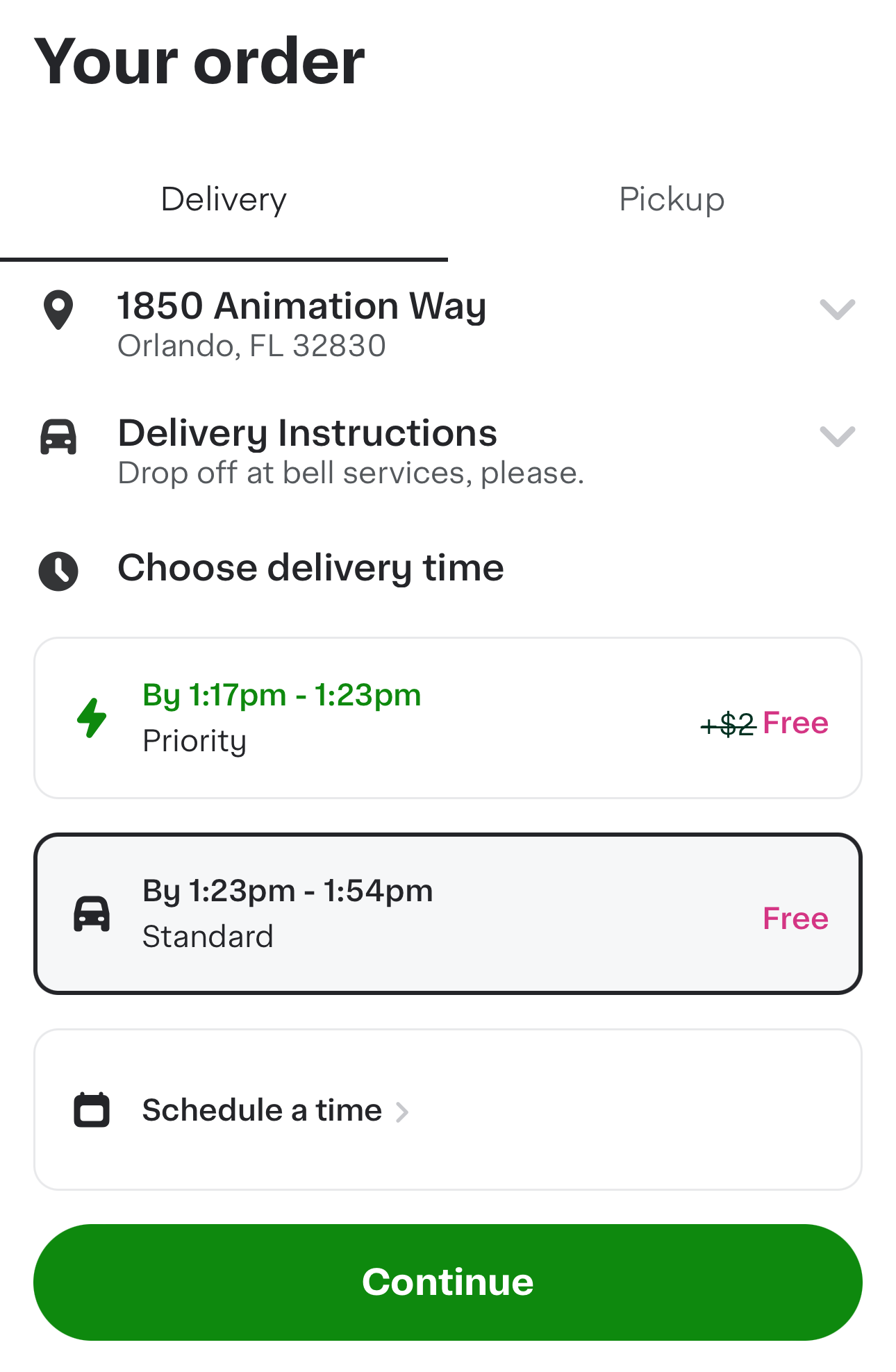The image displays an order confirmation screen with the following details:

At the top of the screen, the title "Your Order" is prominently displayed in black text.

Beneath the title, there are two options for order fulfillment: "Delivery," which is highlighted, and "Pickup," located to the right.

Further down, an address is provided: "1850 Animation Way, Orlando, Florida, 32830."

Below the address, there are delivery instructions that read: "Drop off at Bell Services, please."

Next, the text "Choose Delivery Time" is displayed in black.

Below this heading, there are two delivery time options:
1. The first option, struck through and marked as canceled, shows "By 1:17 PM - 1:23 PM Priority" with a fee of $2, displayed in pink.
2. The second option is highlighted in a black rectangle with a light gray background and shows "By 1:23 PM - 1:54 PM" with a car icon to the left, labeled "Standard" and noted as "Free" on the right in pink.

Further down the screen, there's an option to "Schedule a Time."

At the very bottom of the image is a large, green, oval-shaped button that says "Continue" in white text.